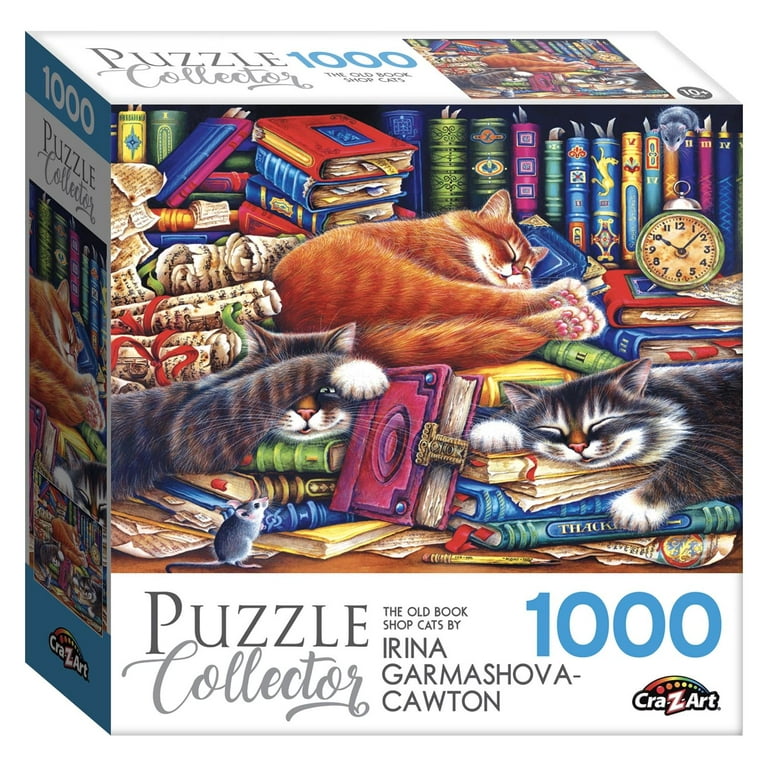The image showcases the packaging for a 1,000-piece jigsaw puzzle by Crazy Art, titled "The Old Book Shop Cats," illustrated by Irina Garmashova Kaltson. The box predominantly features a detailed painted illustration of a cozy personal library. Shelves lined with vividly colored, antique-looking books—complete with bookmarks and notations—are the backdrop. Several rolled-up scrolls, tied with red and green ribbons, complement the setting. In the midst of this scene, three cats with cartoon-like, smiling expressions are napping contentedly among the books. One reddish cat with stripes and white markings is lounging comfortably on its side. A gray, striped cat at the bottom right uses books as a pillow. Another cat, with grayish-brown stripes on the left-hand side, playfully peeks out from under its paw at a small mouse on the table. A second mouse is perched on top of the bookshelf near an old-fashioned clock. The box also has the puzzle's title and artist's name, along with the branding details prominently displayed on the top and sides.